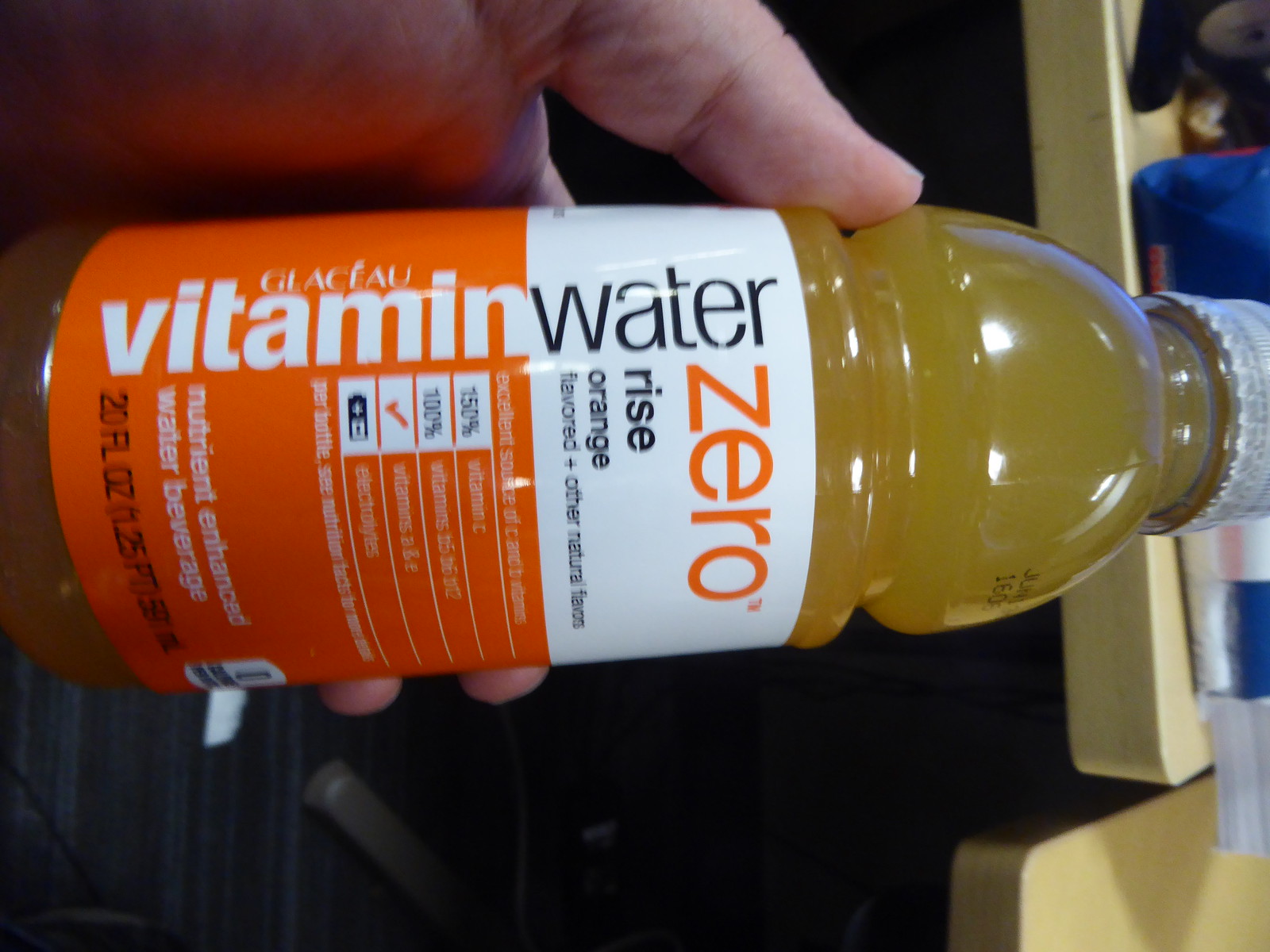This is a photograph of a hand holding a 20 fluid ounce bottle of Glaceau Vitamin Water Zero Rise, an orange-flavored nutrient-enhanced water beverage. The hand is positioned in the upper left-hand corner of the image, with the thumb placed on the bottle and two fingers gripping underneath. The bottle, held horizontally with the clear plastic cap on the right and the base on the left, contains a yellow-orange liquid. The clear bottle features a white label at the top and an orange label on the bottom two-thirds. The text on the label includes "vitamin water" in black and white, "zero" in orange text, and other nutritional details. The background showcases a light beige wooden table with miscellaneous objects, including a blue item and a black object, and a blue carpet on the floor.